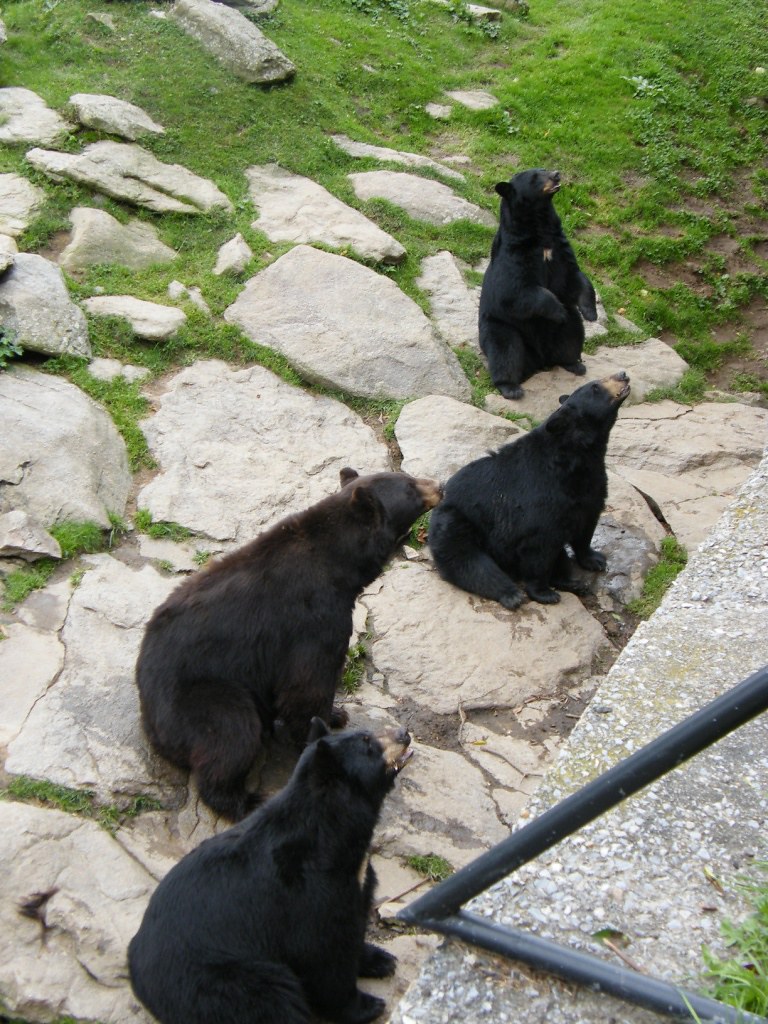This outdoor photograph, likely taken from an elevated viewpoint in a zoo, captures four black bears on a bed of large, flat beige rocks interspersed with patches of green grass. Positioned to the right within the image, all bears are focused intently towards an unseen point to the right, slightly upwards, creating a uniform sense of curiosity or alertness. In the upper section, the terrain transitions from rocks to a grassy area, suggesting a naturalistic enclosure. The central bear, standing on its hind legs, prominently displays a golden marking on its chest, with its front paws raised slightly. To its front lower-left, another bear sits with its head turned up to the right, while a large brown bear to its left gazes in the same direction. In the bottom left, another black bear is seated, also looking to the right. The bears have dark fur with lighter snouts. A black metal pole, embedded in concrete and forming an acute triangular angle, is visible amidst the rocky terrain, adding to the detailing of the enclosure's setting.